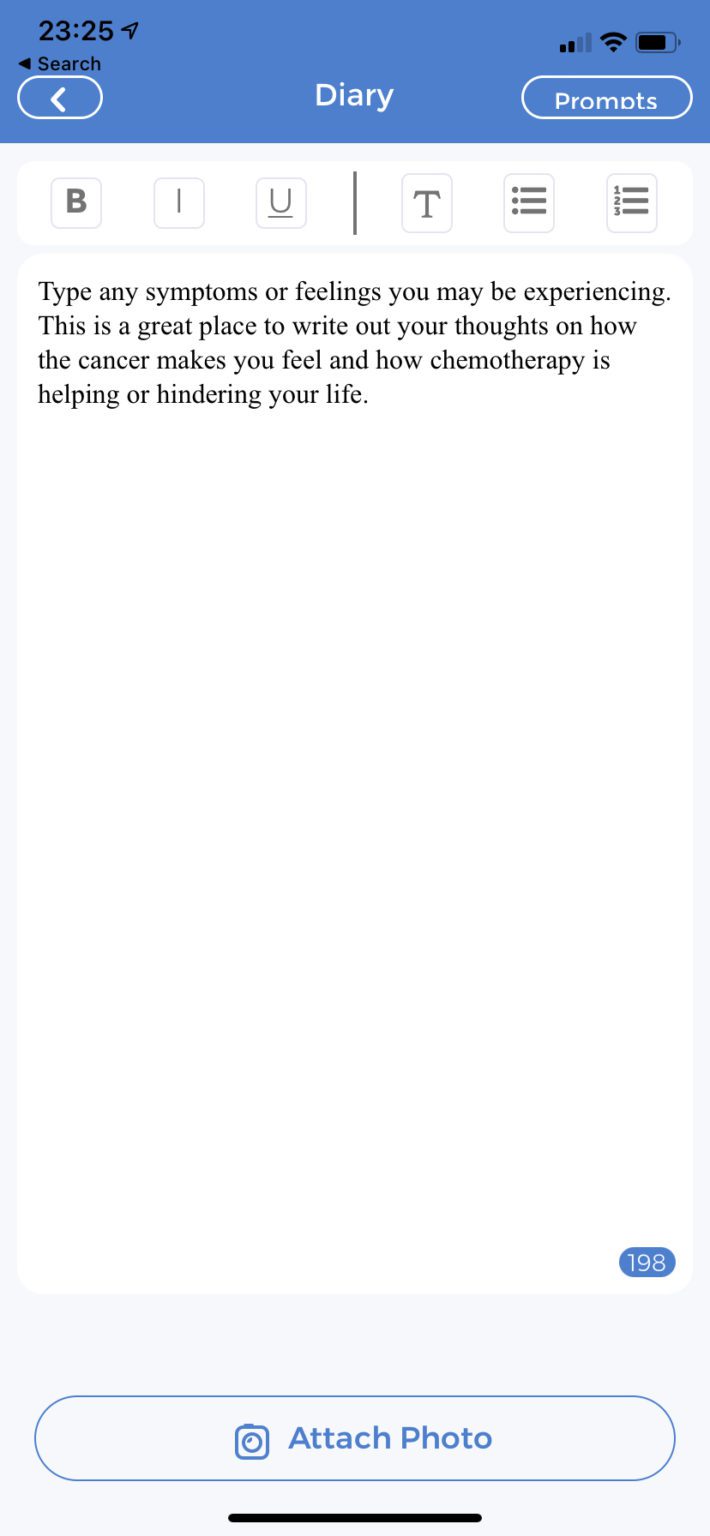A detailed screenshot from a diary app on someone's phone is displayed. 

At the top of the screen, there's a blue header bar. The time "23:25" is visible in the top left corner, followed by a black "Search" label with a left-pointing arrow beneath it. Still within the blue header bar, there's a white oval with another left-pointing arrow. The word "Diary" is centered in white text. To the right, there's another white oval labeled "Prompts" in white text. Above this header, you can see the phone's signal strength and battery life indicators.

Below the header bar, there's a toolbar with various formatting options, presented as gray squares, that allow the user to select bold, underline, and other text formatting options.

Beneath the toolbar, there's a large white vertical rectangle containing black text. The text reads: "Type any symptoms or feelings you may be experiencing. This is a great place to write out your thoughts on how the cancer makes you feel and how chemotherapy is helping or hindering your life." 

In the bottom right corner of this white rectangle, there's a small blue oval with the number "198" written in white inside it. Below this, another vertical blue oval appears with a whitish-gray background. Inside this oval, in blue text, it says "Attach Photo," accompanied by a small camera icon.